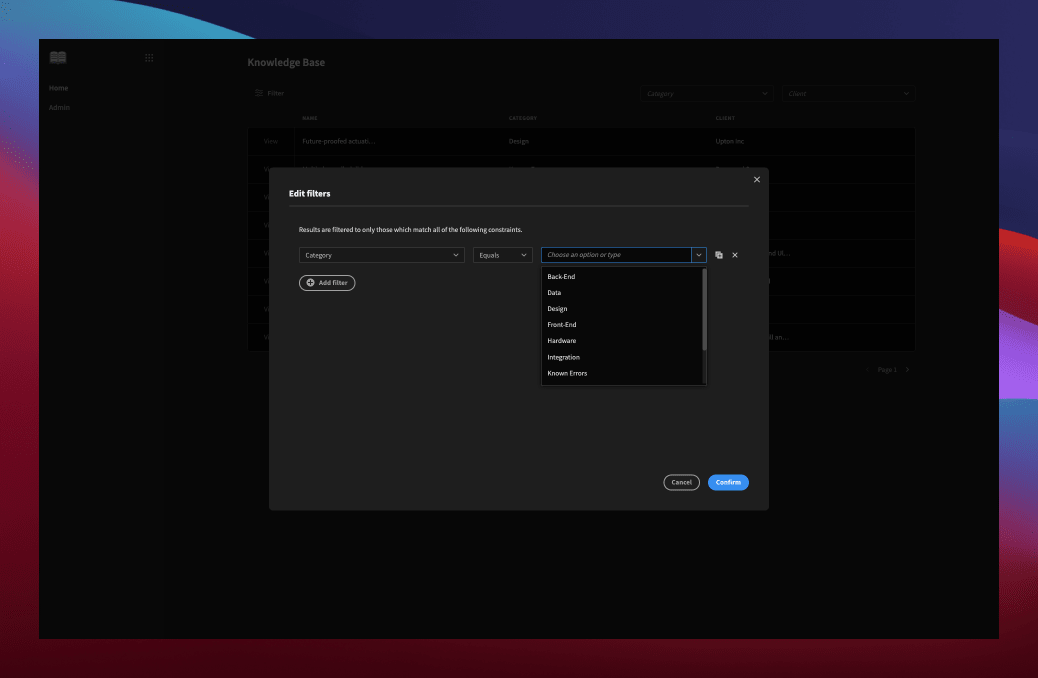**Descriptive Caption:**

The screenshot depicts a website interface in dark mode, primarily showcasing an "Edit Filters" panel. The background of the website is nearly black, slightly grayed out due to the active filter panel. The "Edit Filters" panel is a lighter gray with clear text stating, "Results are filtered to only those which match the following constraints." Below, several dropdown fields are available, such as "Category equals" with selectable options: Backend, Data, Design, Frontend, Hardware Integration, and Known Errors. Despite the small text, these options are visible due to an activated dropdown. At the bottom of the panel, two capsule buttons are present: “Cancel” and “Confirm,” with the latter being a blue button featuring white text. The obscured background displays headings like "Knowledge Base" and several columns, though details are difficult to discern. To the left, a sidebar features an icon of an open book at the top and options labeled "Home" and "Admin."